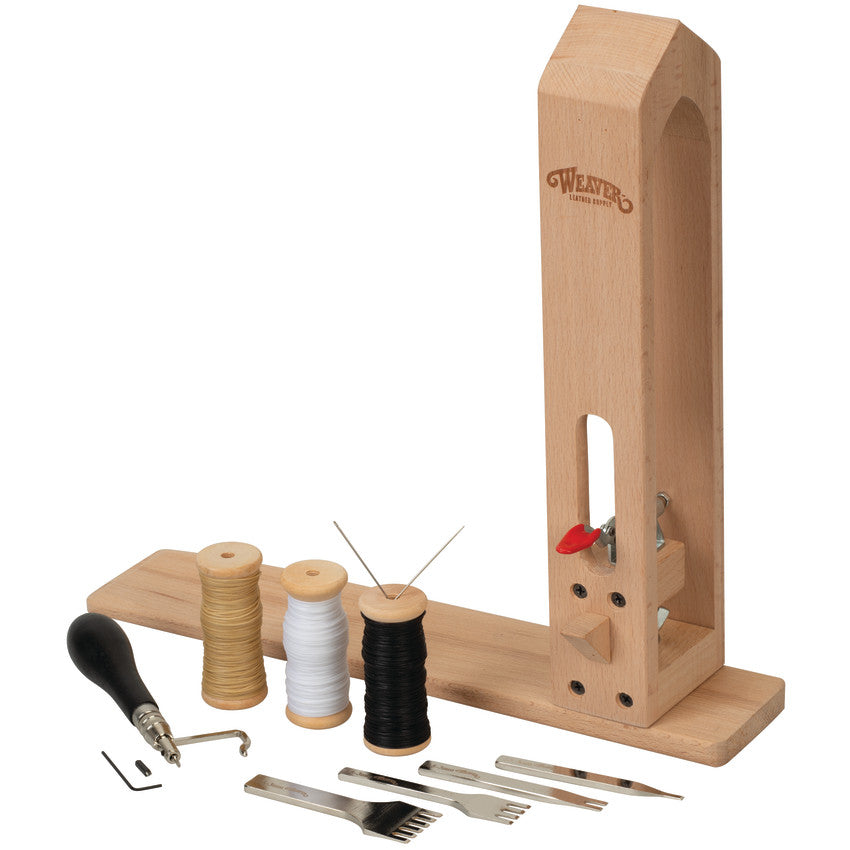This image features a meticulously arranged sewing kit set against a pristine white background. Central to the composition are three spools of thread in brown, white, and black hues, with the black spool prominently displaying two needles inserted into its top. To the right of the spools, a selection of four shiny, silver-colored tools is neatly laid out. These tools appear to be various forms of sculpting or threading instruments, including two that resemble forks, one that has prong-like tips, and another that resembles a pen. Also included is a black tool with a bulbous base and a silver, pointed tip, positioned at the bottom left corner. Behind the spools, there's a wooden base supporting a vertical wooden structure that features an archway cutout and a small red knob protruding from it. Near this arrangement lies a small Allen wrench accompanied by a screw. Overall, the image captures a well-organized array of sewing implements set against a clean backdrop, highlighting both the functionality and aesthetic appeal of the tools.